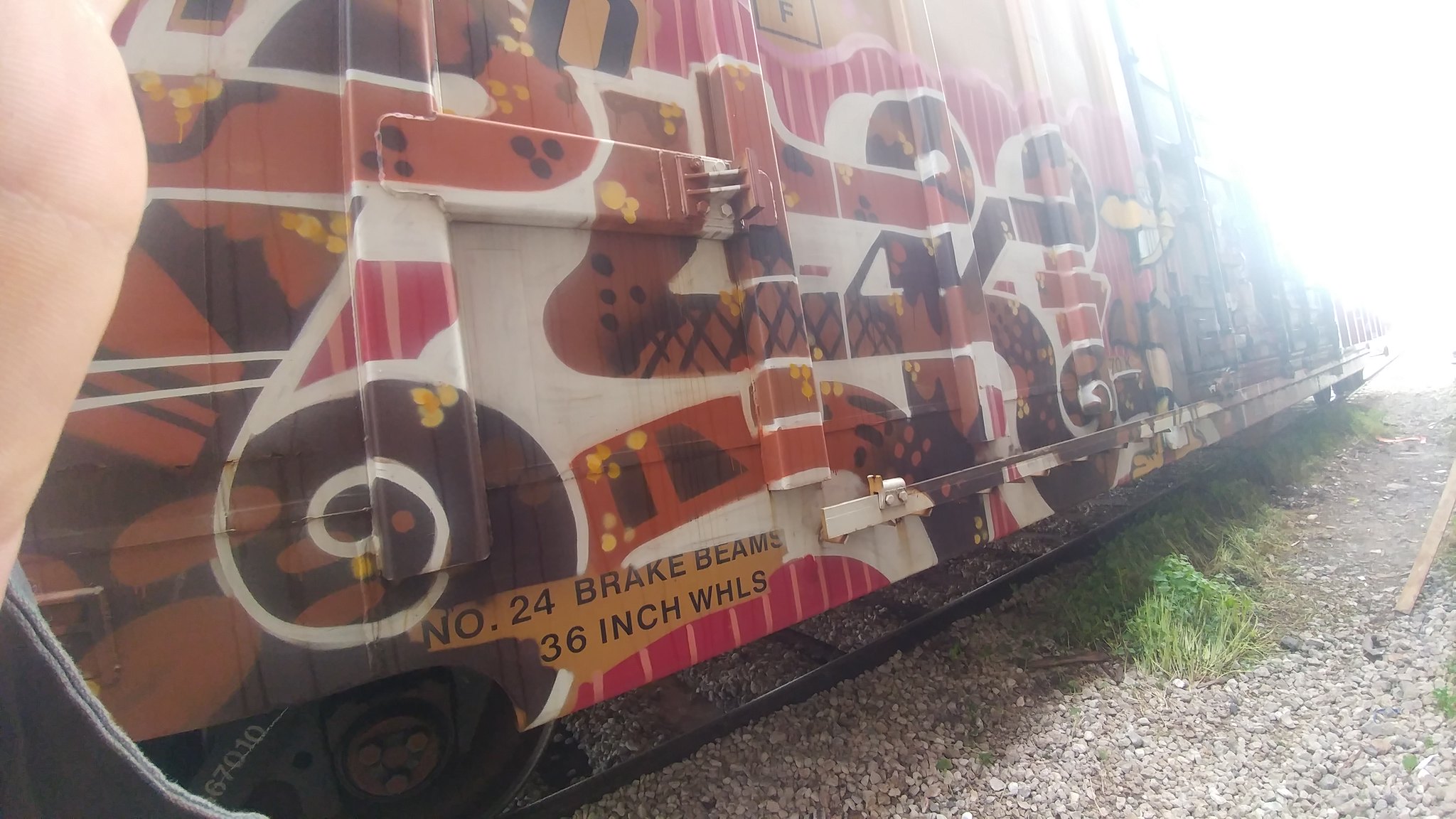The image depicts a blurry train car with a colorful and abstract design, featuring muted tones of brown, dark red, orange, pink, and white, with some shapes appearing as spirals. A part of a person's finger is visible in the top left corner of the photo. The train car bears an orange rectangle with text that reads "No 24 brake beams, 36 inch wheels." The car is positioned on black tracks with gravel underneath, and light green vegetation is sprouting up through the gravel. There is heavy light exposure in one corner of the image, adding to the overall blurriness and giving the impression of a phone with an unclean lens. In the background, other train cars are visible, though they appear blurred.